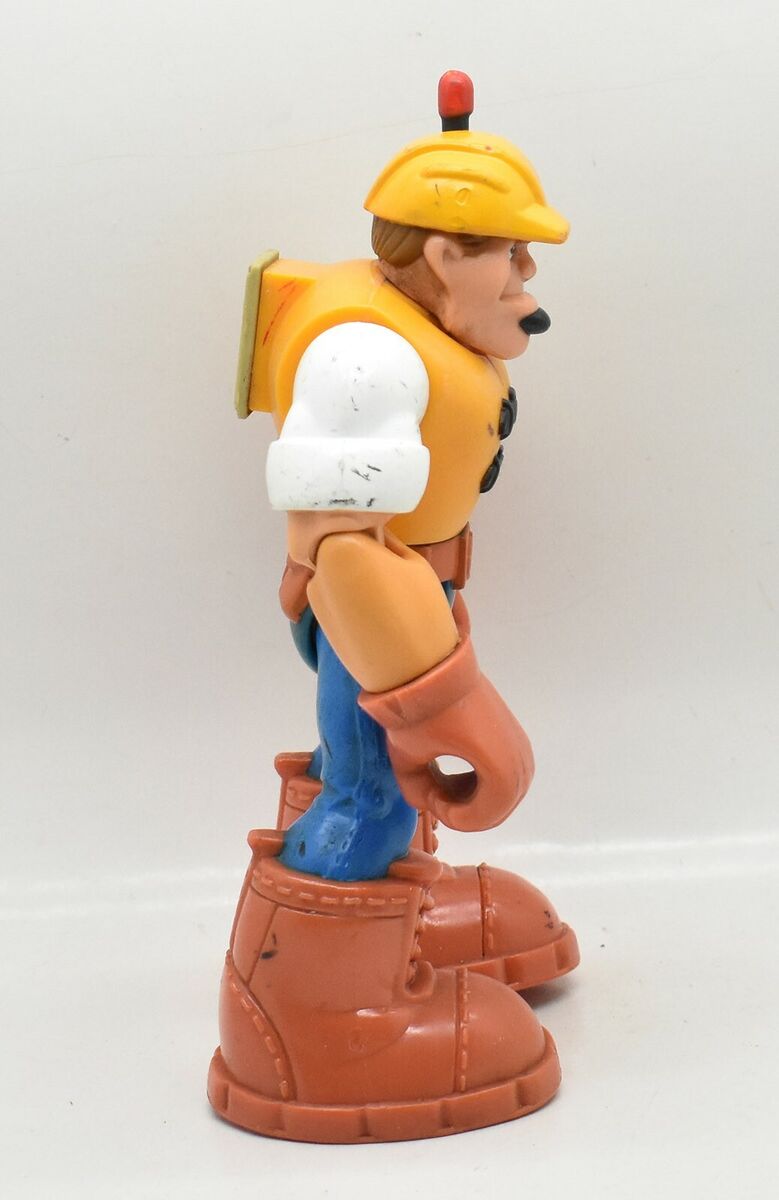This photograph captures a vintage plastic toy figure designed as a construction worker. The figure stands upright on a light gray surface against a light gray background, facing to the right. The toy features large, exaggerated brown boots that shimmer slightly and blue jeans. The figure's arms, which have a hole presumably for attaching accessories, are jointed at the elbows, allowing for movement. 

The toy is detailed with brown gloves and a brown belt. The character wears a white short-sleeved shirt with the sleeves rolled up above the elbows, topped with a yellow vest that has black buttons or fasteners on the front. Additionally, there seems to be a mechanism or possibly a magnet on the back for attachment purposes. The figure's head is adorned with a yellow construction hat and features short brown hair. Notably, an antenna-like object extends from the hard hat, black with a red tip. 

The character has a distinct facial appearance with a prominent chin and a small patch of a beard that doesn't quite match the hair color. Overall, the toy exudes a cartoonish charm with its oversized proportions and detailed outfit, suggesting it is part of a larger set or system of toys.